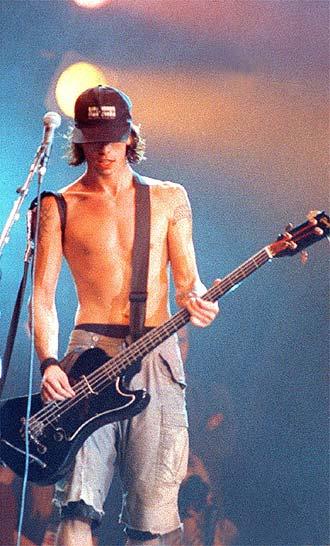In this image, the focal point is a shirtless man positioned directly in the center, holding a black guitar, and standing before a microphone. The backdrop, a dimly lit and somewhat hazy room, casts an enigmatic atmosphere with lights visible in the upper left corner. The color palette we can discern includes shades of blue, white, yellow, orange, black, silver, tan, and hints of pink. The man, described as long and tall, wears a black hat with brown hair peeking out from under it, his head slightly bowed so his eyes are obscured. The microphone extends up the left side of the image, appearing as tall as he is and aligning with his head. Trailing from his acoustic performance, the guitar strap traverses his chest, leading down to his light blue cutoff shorts with visible pockets. The grainy texture of the background adds to the image's raw and unrefined feel, suggesting an indoor or outdoor concert setting.